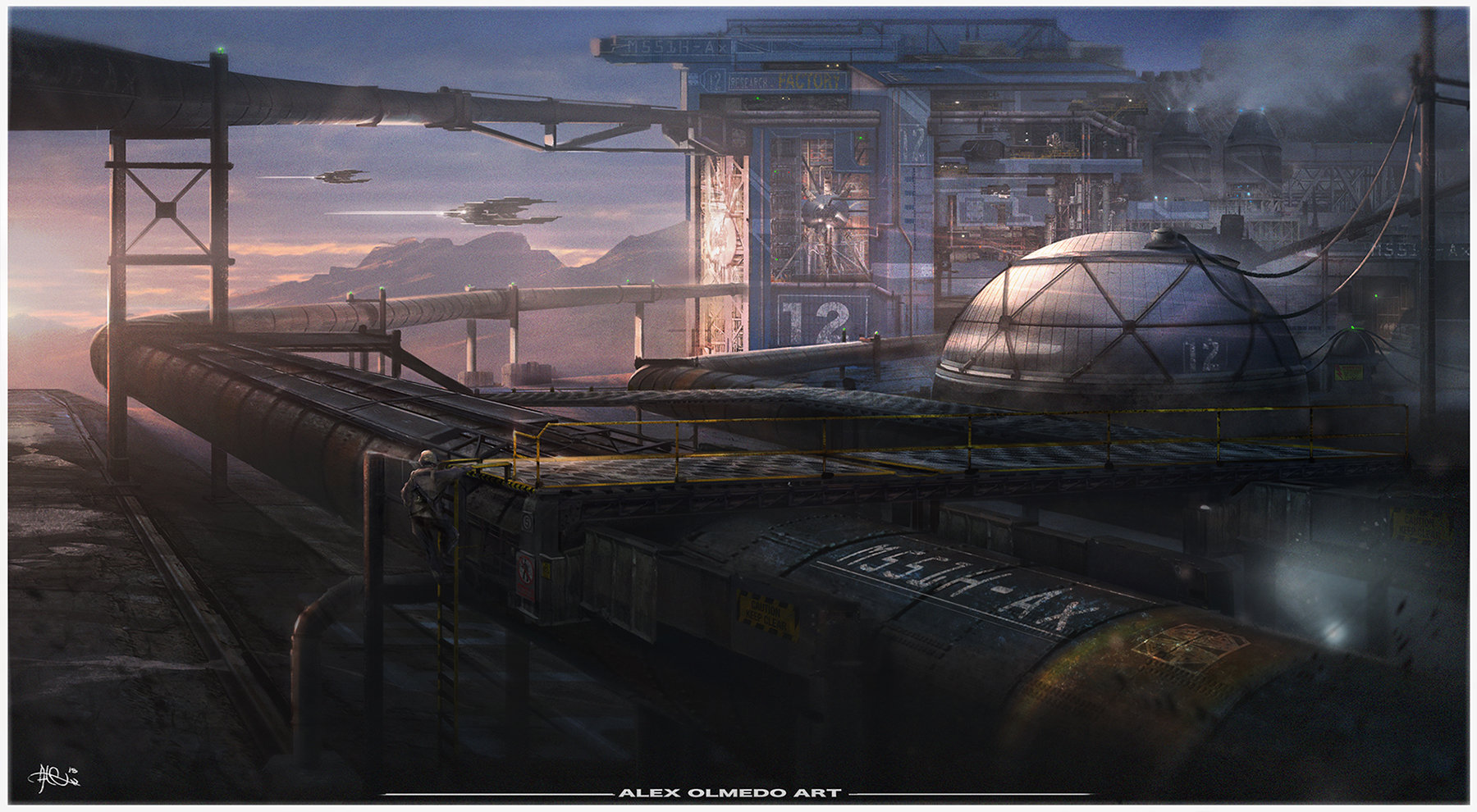The image appears to be a detailed and intricate piece of futuristic artwork, attributed to Alex Almeydo, as indicated by the white text "Alex Almeydo Art" at the bottom. The scene depicts a dystopian metropolis infused with an industrial and futuristic aesthetic. Central to the image is a large building marked with the number "12," accompanied by another similarly numbered structure and a domed building displaying the same digit. Adding to the dystopian feel, there are big, tube-like pipes and a network of tunnels with one labeled "M537H-AX." The cityscape is enveloped in a palette of gray, white, black, yellow, purple, pink, and blue hues, with smoke and telephone wires accentuating the gritty ambiance. Spaceships with lights hover above, suggesting an advanced, possibly dystopian future. The rendering might be from a video game, indicated by the absence of people or organic matter, and the setting conveys a slightly darker tone, possibly during sunset or sunrise. The artwork could be a watercolor or oil painting, resonating with a futuristic, industrial complex in a modern, dystopian world.